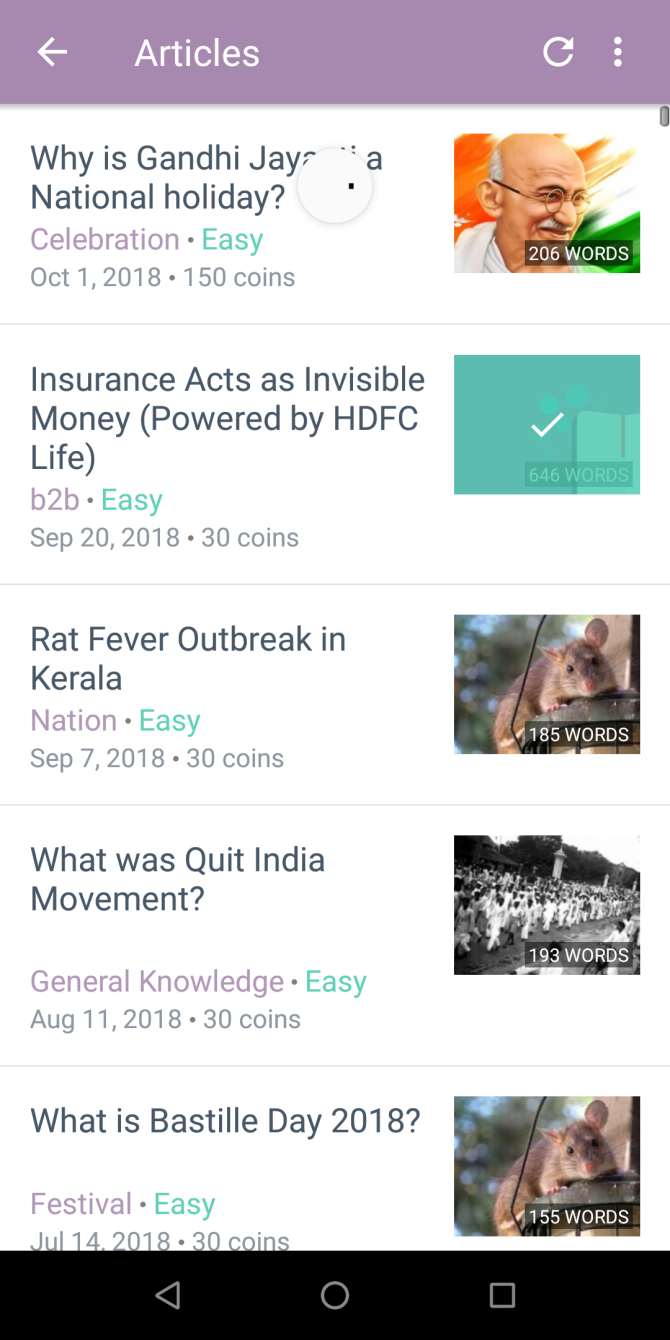The image is a screenshot captured on a mobile device displaying a news application interface. At the very top of the screen, there is a prominent purple bar with the title "Articles" written inside. Directly below this title are five listed articles, each presumably clickable, indicating their interactive nature. The articles presented in order are:

1. "Why is Gandhi a National Holiday?"
2. "Insurance Acts: Why Insurance Acts as Invisible Money"
3. "Rat Fever Outbreak in Kerala"
4. "What Was the Quit India Movement?"
5. "What is Bastille Day 2018?"

Each of these headlines suggests informative content, addressing various historical, economic, health-related, and cultural topics.